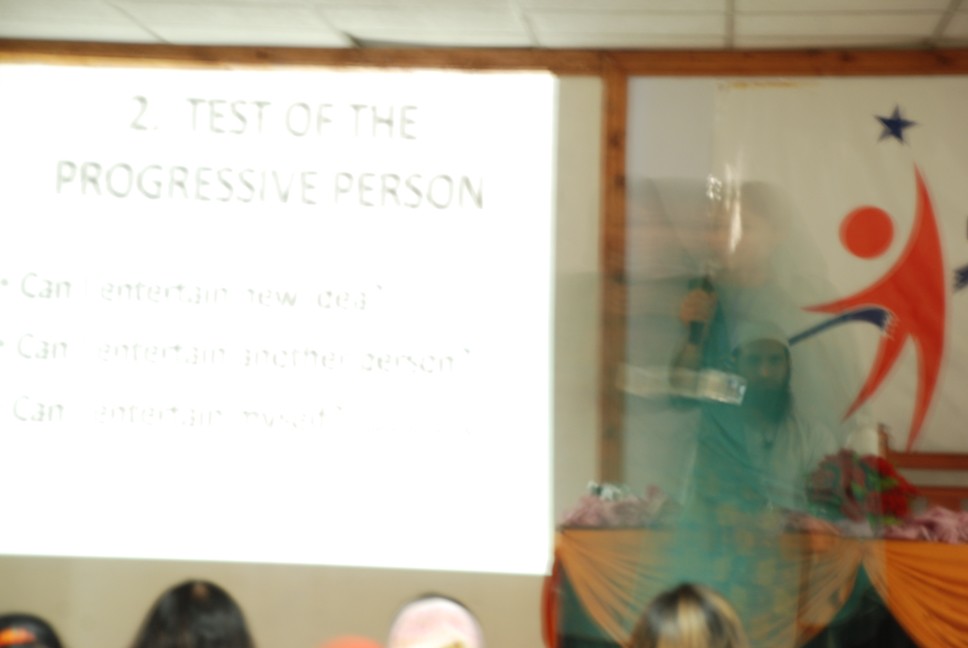In the photograph, a classroom setting is depicted. The upper part of the image showcases a white drop ceiling, characterized by white tiles and tan-colored dividers. Just below the ceiling, there is a prominent horizontal strip of wood, with a reddish-orange hue and noticeable black knots. At the center of this strip, a vertical piece of the same wood extends downward, dividing the visual space.

Flanking this central vertical piece are two whiteboards. On the left side of the image, a notable bright white square is mounted on the whiteboard. This square features light black text at the top, reading "TO TEST OF THE," followed by "PROGRESSIVE PERSON" in all capital letters. Additional black writing is visible beneath these headings.

The bottom of the photograph captures the top rear view of several peoples' heads, suggesting an audience or classroom attendance. On the right side of the whiteboard, various colorful shapes are displayed: a red circle, a red triangle with three extending tentacle-like lines, and a blue star, adding a vibrant touch to the scene.